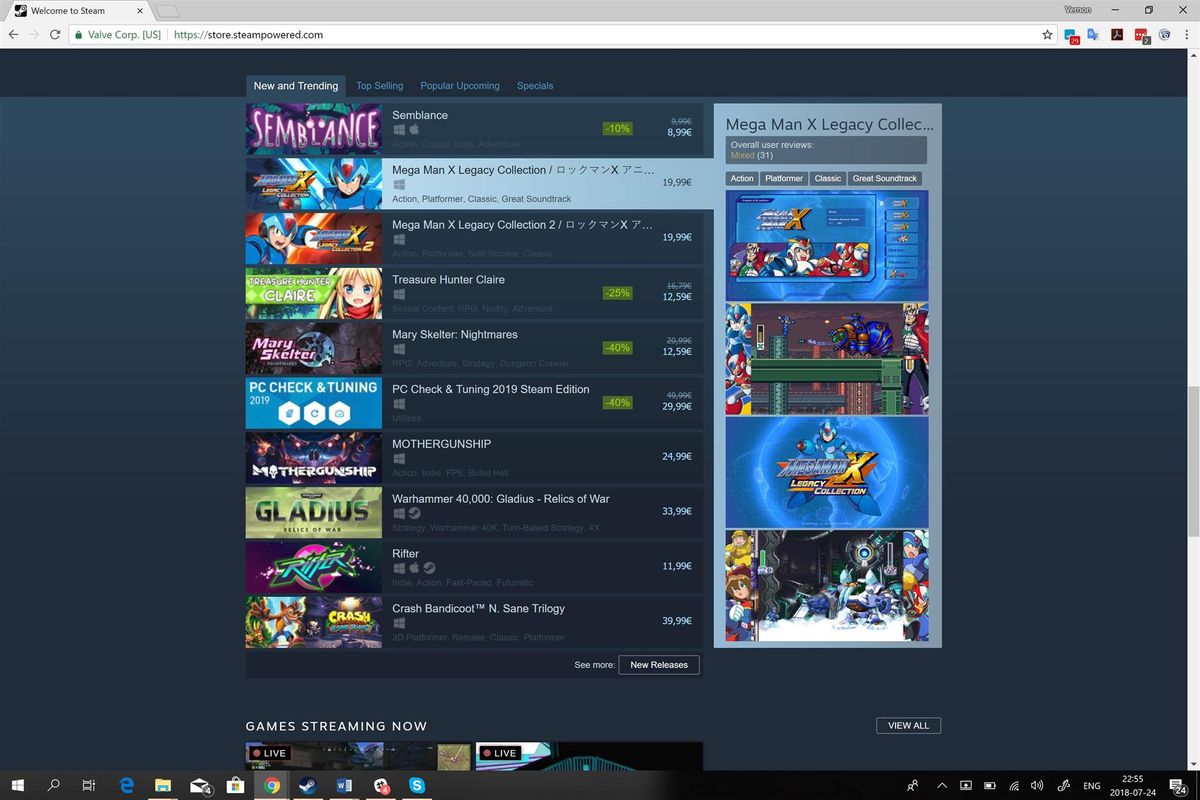In this image, a user is browsing the Steam website, specifically the 'News and Trending' section. The top left corner of the website displays the Steam logo with the text "Welcome to Steam," and the URL is shown as "store.steampowered.com." Steam is an online platform where users can find and purchase various video games, some of which are free while others require payment or a membership.

At the top of the website, there are several categories including 'Store,' 'News and Trending,' 'Top Selling,' 'Popular Upcoming,' and 'Specials.' The user is currently focused on the 'News and Trending' section. This section displays both graphical artwork and video previews of different video games.

The first game featured is "Semblance," which is available for both Windows and Apple platforms. It is currently on a 10% discount, reducing its price from €9.99 to €8.99, indicating the user is viewing the European version of the store. The game’s genre and age rating are also mentioned but are hard to read in this image.

Following "Semblance," the next game shown is "Mega Man X Legacy Collection," priced at $19.99, and available exclusively for Windows. The game is tagged as an action platformer and is praised for its classic gameplay and great soundtrack. Another title, "Mega Man X Legacy Collection 2," is depicted similarly, also priced at $19.99.

Additional games such as "Treasure Hunter Claire" and "Mary Skelter: Nightmares" are listed, along with a few others. At the bottom of the list, there is an option to "See More" which leads to new releases.

To the right of the "Mega Man X Legacy Collection" listing, there are several screenshots of the game, allowing users to preview the gameplay. The game's user reviews are displayed as well, revealing a mixed rating based on 31 reviews, providing insights into the overall reception by the community.